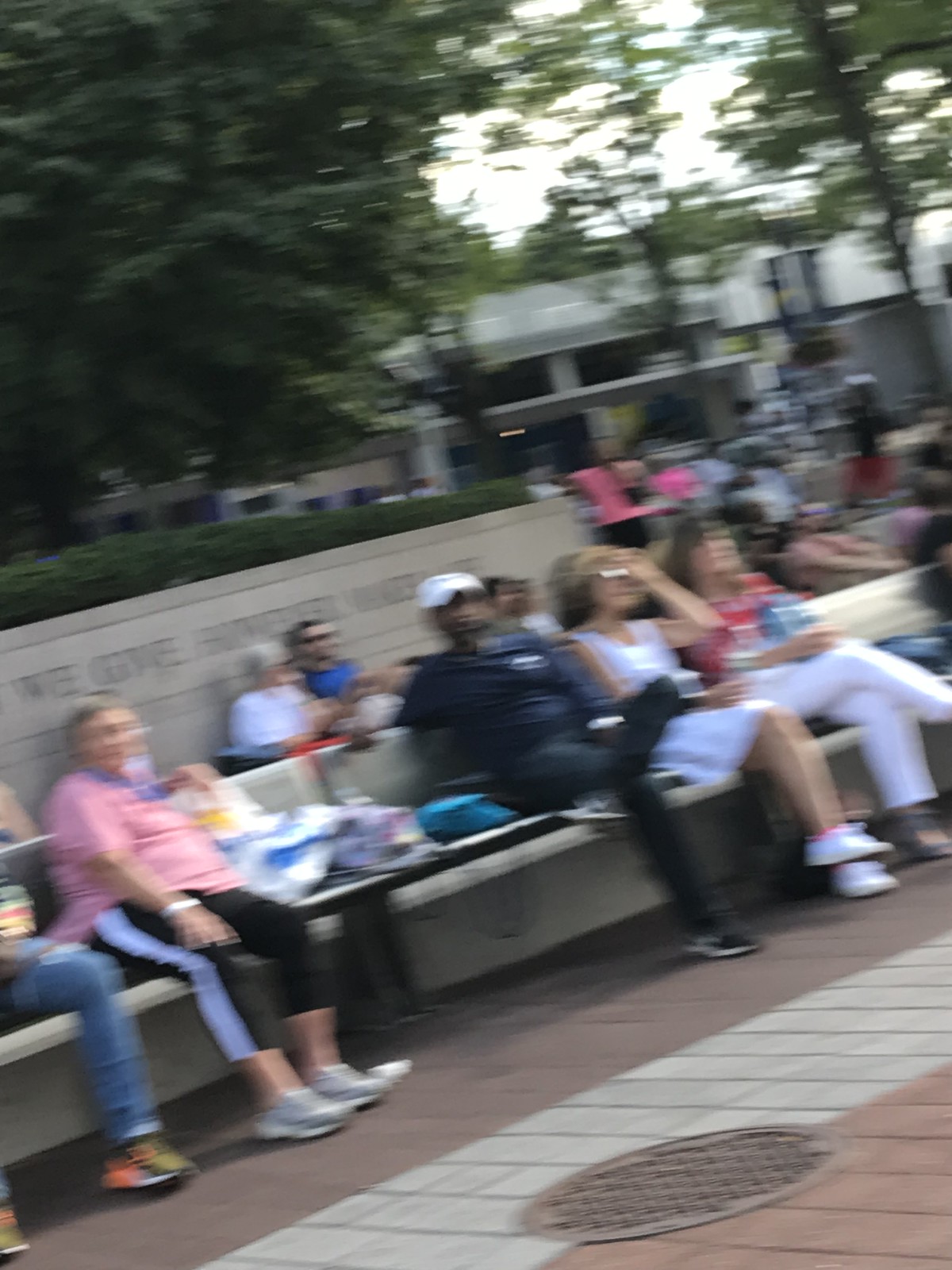This outdoor photograph, slightly taller than its width, captures a serene yet bustling scene, despite its blurred quality. In the lower right corner, a brick pathway is visible, intersected by a metal grate. Stretching diagonally from the lower left to mid-right is a stone or concrete seating area, upon which five individuals are casually seated. Behind them, there is another seating ledge, adjacent to a wall. The wall, adorned with the barely legible phrase "We Gave and [unreadable]," has a grayish tone. A lush green tree, bathed in shadows, stands behind the seating, while a portion of the sky peeks through an opening in the upper right corner. In the background, a gray building extends towards the right, completing the ambient urban landscape.